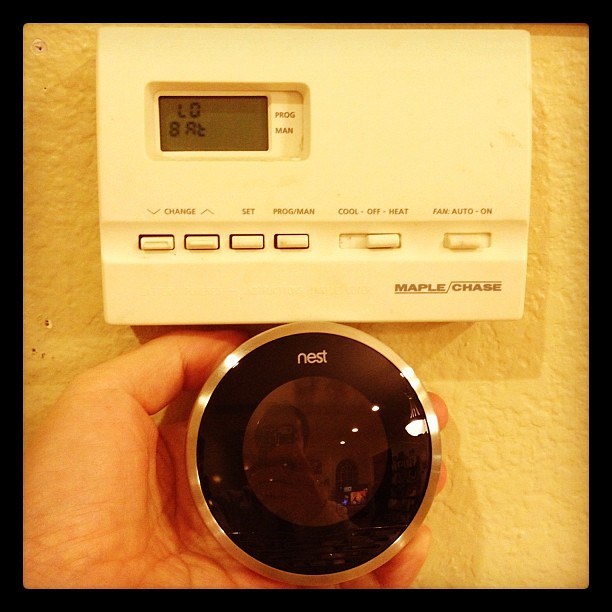This portrait-style photograph captures a detailed view of a thermostat and a Nest camera positioned below it, mounted on a cemented white wall bathed in a warm, yellow light. A hand extends from the bottom left corner of the image, wrapping around the back of the Nest camera. The Nest camera itself is circular with a sleek silver outline, featuring a larger black circle in the center and a smaller purple lens at the very center. The word "nest" is prominently displayed in white at the top of the black circle. The camera's reflective surface shows a man with short black hair holding a phone, obscuring his face, with his fingers clearly visible around the black phone's edge.

Above the camera, the thermostat is a white, horizontally shaped rectangle with a small LED screen positioned to the left. The display reads "LO8AT," while the right side features the words "prog" and "man" in gray. Below the display, there are six buttons labeled as follows: "change" with up and down arrows beside it, "set," "program/man," "cool-off-heat" (set to heat), and "fan auto/on" (set to auto). Each element is meticulously detailed, offering a comprehensive view of the devices and their settings.